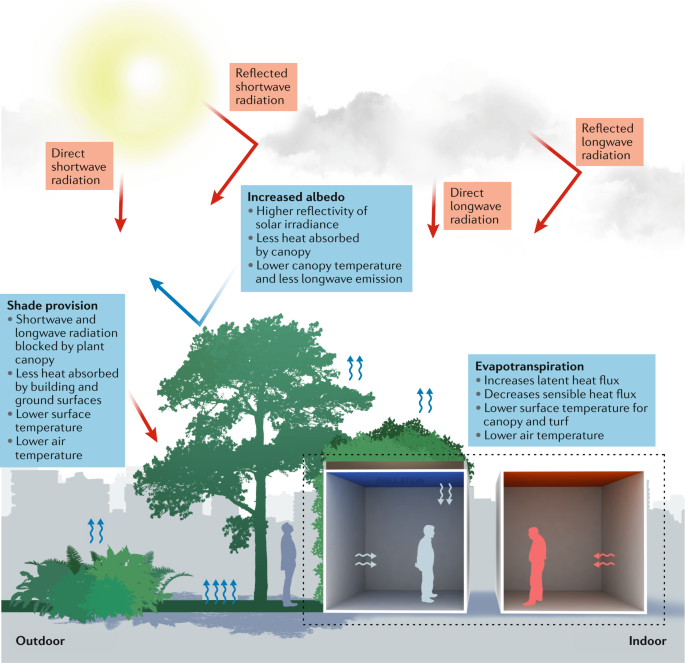This infographic illustrates the mechanisms of shortwave and longwave radiation, emphasizing their interaction with plant canopies and their role in regulating temperature. On the left side, the sun is depicted with an orange box labeled "direct shortwave radiation," accompanied by a red arrow. Nearby, another orange box labeled "reflected shortwave radiation" features an arrow with a 90-degree bend. Below, a blue rectangle explains "shade provision," detailing how plant canopies block both shortwave and longwave radiation, resulting in lower heat absorption by buildings and ground surfaces, which leads to lower surface and air temperatures. 

In the middle, closer to the top, another blue rectangle highlights "increased albedo"—the higher reflectivity of solar irradiance by plant canopies, which reduces heat absorption and lowers canopy temperature while decreasing longwave emissions. Adjacent to this, arrows pointing right indicate "direct longwave radiation" and "reflected longwave radiation" in orange boxes.

At the lower section is a visual showing greenery, including a tree and bushes, with people situated inside and outside structures. The left structure has a blue ceiling with grass on top, indicating lower temperatures, while the right structure has a red ceiling, symbolizing higher temperatures. The graphic clarifies indoor and outdoor conditions, demonstrating how shade and plant presence reduce heat. Additionally, text near the bottom right explains "evapotranspiration," describing its role in increasing latent heat flux, decreasing sensible heat flux, and consequently lowering surface and air temperatures. The combined elements underscore the importance of plant canopies in mitigating heat and enhancing human comfort.